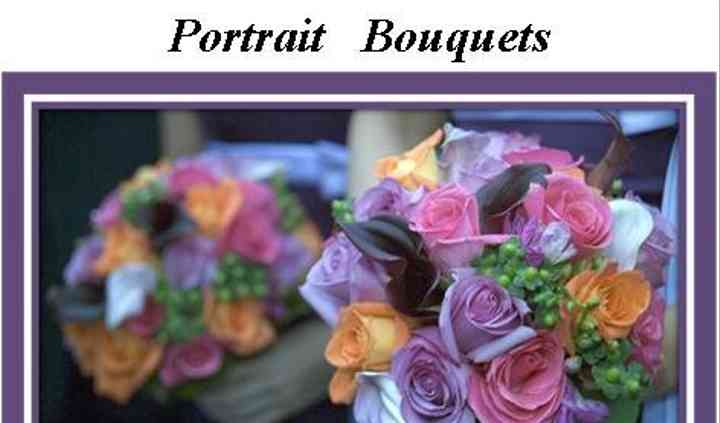The image showcases an elegant arrangement of flower bouquets, primarily featuring lilac purple, light pink, light orange, and white roses accented by dark green or black leaves and sprigs of greenery. The photograph is adorned with a partially completed purple and white frame, suggesting that the bottom portion of the image may be cut off. The bouquet on the right side of the image is prominent, with a person’s hand clearly visible, holding the flowers. This bouquet includes lavender, peach, and dusty pink roses, all nestled within the greenery. A blurred second bouquet appears in the background on the left, mirroring the primary bouquet's composition. The entire scene is framed above by black text reading "portrait bouquets," indicating the image might be part of an advertisement. The overall setting suggests a dignified ambiance, like one associated with Mosques or grave sites, with a feeling enhanced by the cemented bowl-like container typically seen in such places. The blurred background provides an additional depth, making the front bouquet stand out even more.